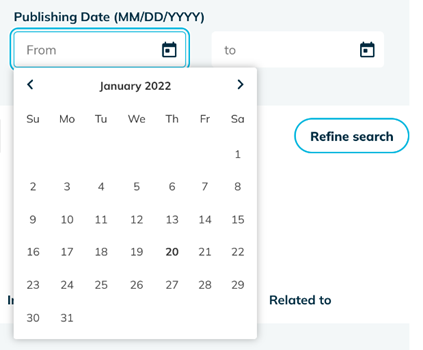The image features two layered screens. The larger, original screen serves as the backdrop, with a smaller overlay page positioned above it. The top of the original screen is adorned with a light gray-blue banner that spans its width. Within this banner, positioned at the top, there is black text that reads: "Publishing Date (MM/DD/YYYY)".

Beneath the banner, there is a white box outlined in light blue. This box contains gray placeholder text that reads "From," accompanied by a calendar icon on its right side. Adjacent to this is another white box that bears the gray text "To" on the left, also featuring a calendar icon on the right.

In front of these elements, a calendar pop-up is displayed. The header of the calendar reads "January 2022" in black text, flanked by back and forward navigation arrows. Below the header, the days of the week are listed in a row, starting with Sunday and followed by Monday, Tuesday, Wednesday, Thursday, Friday, and Saturday.

The calendar grid shows that January 1st falls on a Saturday. The date January 20th is highlighted in black, distinguishing it from the other dates, which appear in a lighter gray hue.